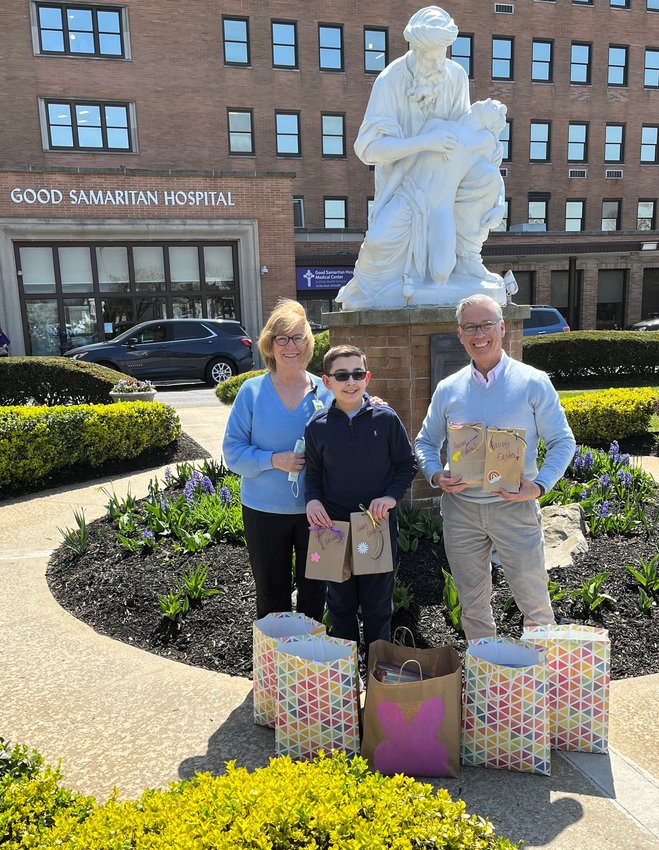The image depicts three individuals standing in front of a statue outside the Good Samaritan Hospital, a large old brick building with many windows. The statue, with an ancient look, portrays a person holding onto another. The people include a young boy with short brown hair, wearing a blue jacket, blue pants, and sunglasses, holding two brown paper bags adorned with "Happy Easter" and ribbon loops. To the boy’s left stands an older gentleman with gray-white hair, a gray sweatshirt, and light-colored pants, also holding two similar paper bags. On the boy’s right, a woman with shoulder-length blonde hair wearing a blue shirt and holding a mask in one hand has her other hand resting on the boy's shoulder. Several large gift bags, featuring an Easter bunny design and a rainbow tile pattern, are placed at their feet. The scene is set on a round sidewalk surrounded by shrubs, with cars parked nearby, indicating they are likely preparing to distribute Easter-themed goodies.